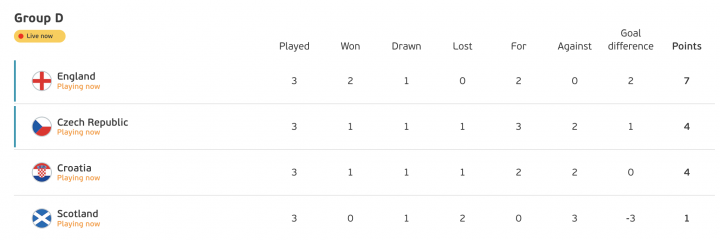The image depicts the standings of Group D in a sports tournament, showing current results. At the top left, the heading "Group D" is prominently displayed. Below this heading, there is a yellow oval with the text "Live Now," indicating that the game is currently in progress. The teams listed are England, Czech Republic, Croatia, and Scotland, each with specific statistics aligned in columns. 

The columns from left to right are labeled: Played, Won, Drawn, Lost, For, Against, Goal Difference, and Points. The numerical data for each team is as follows:

- **England:** 3 matches played, 2 won, 1 drawn, 0 lost, with 2 goals for, 0 goals against, a goal difference of +2, and 7 points.
- **Czech Republic:** 3 matches played, 1 won, 1 drawn, 1 lost, with 3 goals for, 2 goals against, a goal difference of +1, and 4 points.
- **Croatia:** 3 matches played, 1 won, 1 drawn, 1 lost, with 2 goals for, 2 goals against, a goal difference of 0, and 4 points.
- **Scotland:** 3 matches played, 0 won, 1 drawn, 2 lost, with 0 goals for, 3 goals against, a goal difference of -3, and 1 point.

The background of the image is a plain white color, with black bars next to the names "England" and "Czech Republic" for emphasis or highlighting.